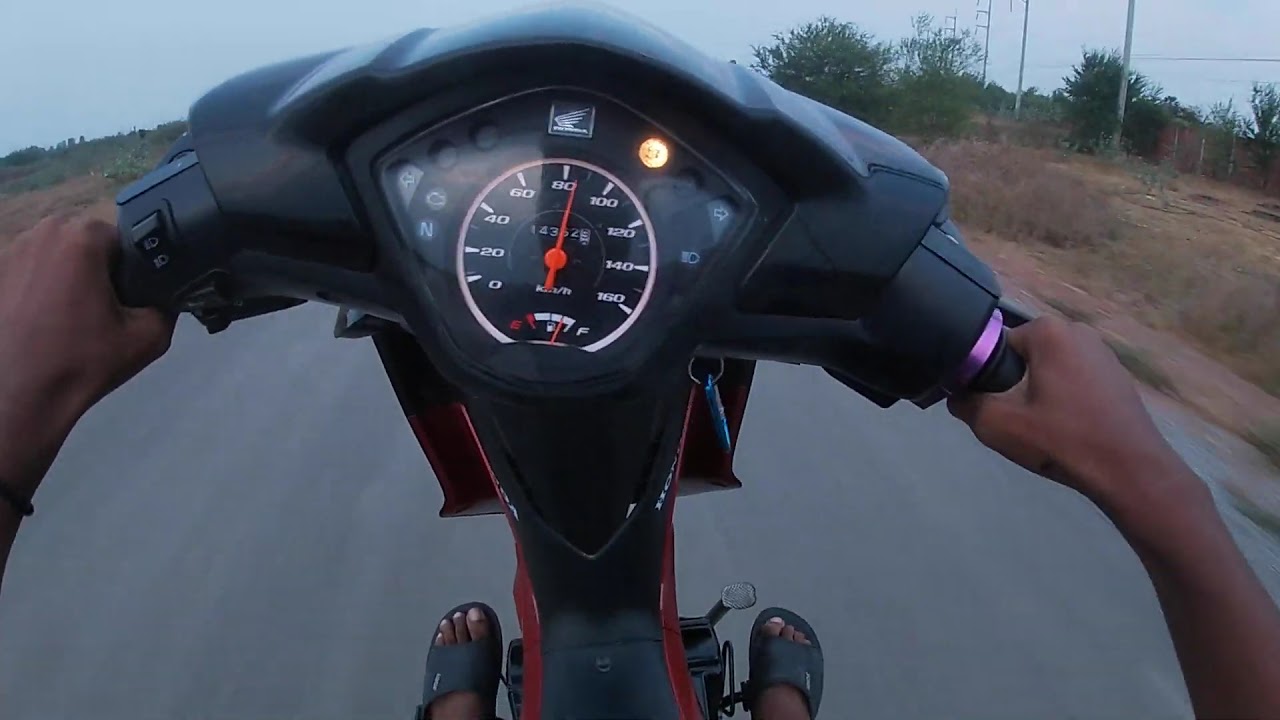The image depicts a close-up view from the perspective of someone driving a scooter down a paved, gray roadway. The focus is primarily on the red and black scooter's dashboard, which features a diamond-shaped console with a circular speedometer showing nearly 85 miles per hour. The rider's dark brown hands grip the handlebars, and their feet, adorned in black sandals, rest on the scooter's base. The scooter displays an eagle wing emblem. The surrounding environment includes a dull, gray sky with some trees and telephone poles visible on the right side. The roadside features a mix of dry, brown grasses and some scrubby brush, as well as a wooden fence. The scene appears to be at dusk, with low lighting conditions contributing to the muted tones. There are no words or text visible in the image.